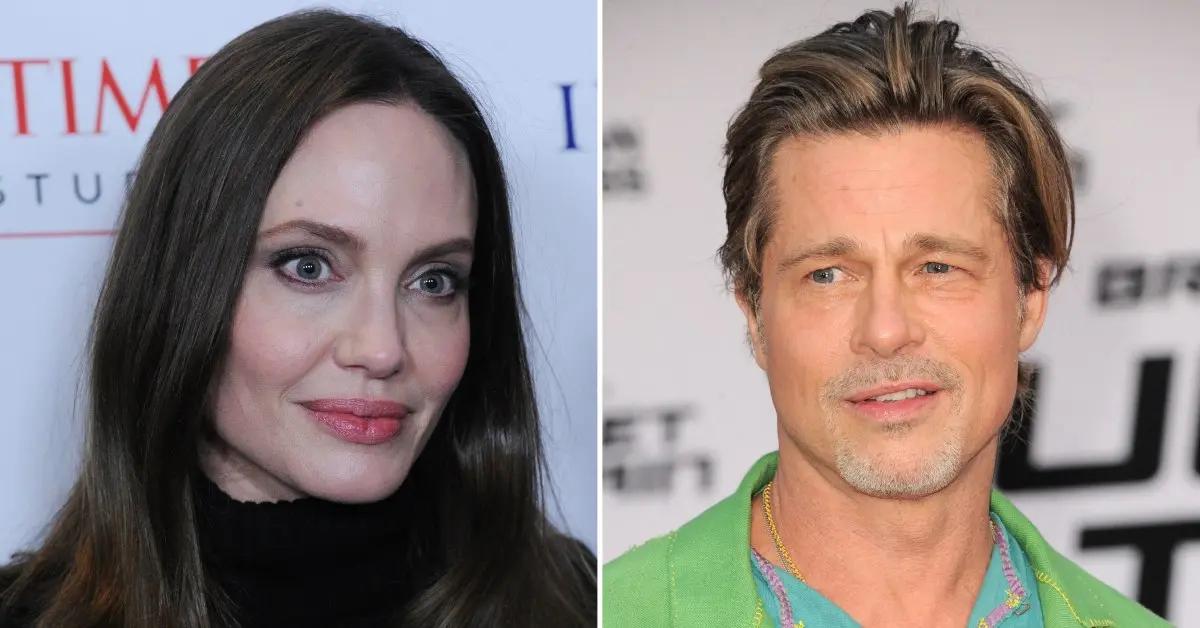In this composite image, we see two side-by-side color photographs of famous actors Angelina Jolie and Brad Pitt, both captured in head and shoulder views. Angelina Jolie is on the left, sporting long, dark brown hair parted in the middle and cascading just past her shoulders. She has blue or dark eyes, is wearing natural-looking makeup with mascara, eyeliner, and pinkish or red lipstick. Her attire is a simple black turtleneck, and her expression is subtly amused with a slight, closed-mouth smile. Behind her is a white background with the distinct red "TIME" lettering, reminiscent of a magazine cover.

On the right is Brad Pitt, appearing with light brown or dirty blonde, slicked-back hair and a gray goatee that complements his casual, slightly smirking demeanor. He wears a vivid lime green jacket over a turquoise or teal shirt with contrasting pink seams, accessorized with a visible gold chain necklace. His gaze is directed slightly to the left, and a partial backdrop with illegible black text suggests a formal event. The combination of their photo's composition, attire, and nuanced expressions provides a contemporary, candid glimpse of these well-known personalities.